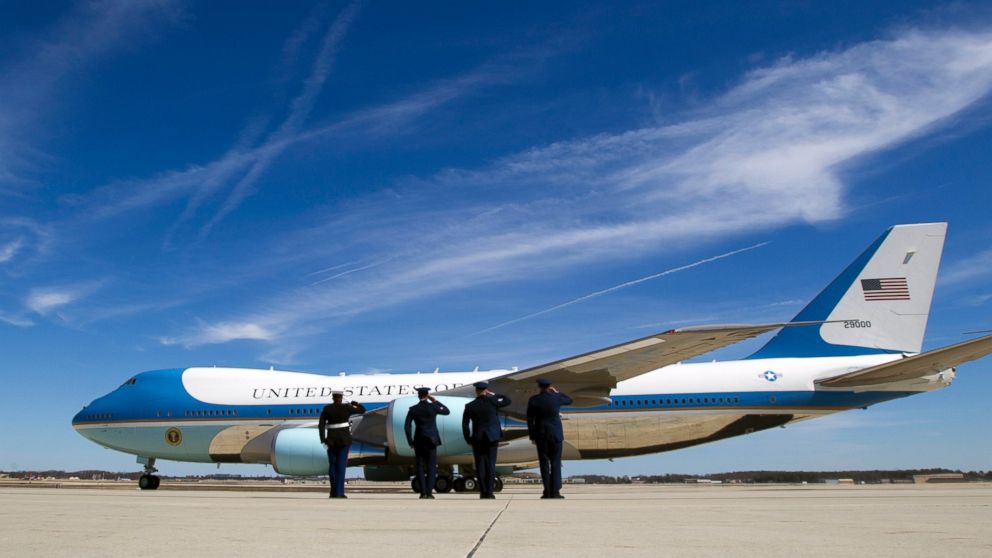This color photograph captures Air Force One stationed on a concrete tarmac, framed by a clear blue sky with wisps of white clouds and faint airplane trails in the upper right corner. The iconic aircraft, predominantly white with a blue nose and a blue stripe running along its midsection, has "United States of" visible on its side, though "America" is obscured by the plane's wing. Near the front, the presidential emblem is prominently displayed. The tail is decorated with the American flag and the identifier 29000. In formation on the tarmac, four soldiers in dark uniforms stand at attention, saluting the majestic plane. The scene is both orderly and patriotic, encapsulating the solemnity of their duty.